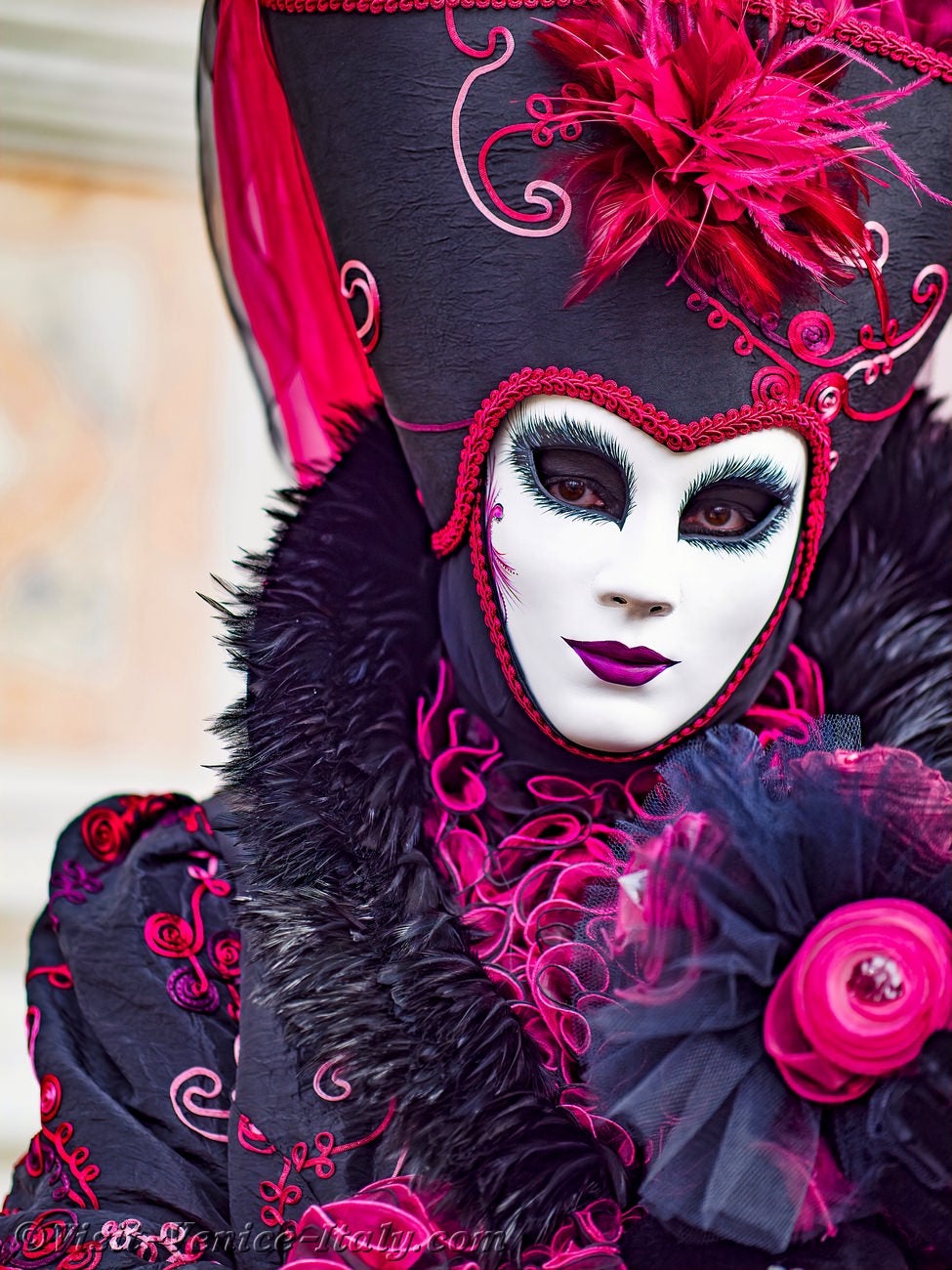In the bustling scene of what appears to be a Mardi Gras parade or perhaps a vibrant celebration, a striking figure stands out, possibly a woman, adorned in a captivating and elaborate costume. Her face is partially obscured by a stark white mask reminiscent of the Phantom of the Opera, which frames her eyes, highlighted with green accents. Below the mask, her lips are painted a deep, bold purple. Crowning her head is a magnificent, oversized black hat that forms a heart shape around her face, festooned with intricate designs and lush pink feathers.

The costume is a splendidly extravagant affair; she wears a grand jacket in black, interspersed with fuchsia pink that complements the vivid feathers of her hat. A flamboyant boa drapes around her neck, adding to the lavishness of her look, while a prominent pink flower with black petals decorates her chest. The sleeves of her attire are long and intricately designed with pink and red swirls that mimic the appearance of flowers. The overall ensemble exudes an air of joyous festivity, embodying the colorful and celebratory spirit of Mardi Gras or a similar exuberant occasion.